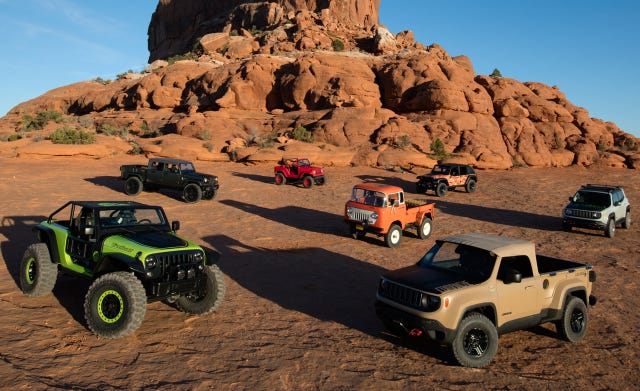This vibrant and detailed image captures a rugged desert scene, likely set in the southwestern United States, such as Arizona, New Mexico, or Colorado. The focal point is a collection of six nearly identical off-road vehicles, all parked in a loose circle against a backdrop of large red rock formations resembling a mountainous plateau. The terrain is characteristic of desert conditions, with dark brown sandy ground and sparse scrub brush, under a bright blue sky.

At the center of the circle is an old-fashioned orange pickup truck, flat-fronted and seemingly from the 1940s, with hay in its bed. Surrounding this centerpiece are various colorful vehicles: a lime green 4x4 Jeep with big tires partly visible on the left, a black Jeep pickup truck next to the green one, and a red Jeep with black tires and red spokes, which is topless and features just a roll bar. There is also a beige Jeep with a black hood and a modern tan Jeep Renegade with black tires and wheel wells on the right, alongside another dune buggy-like vehicle that has a woody appearance with red and yellow accents on its doors and fenders. Each vehicle stands out vividly, adding to the dynamic composition of the scene.